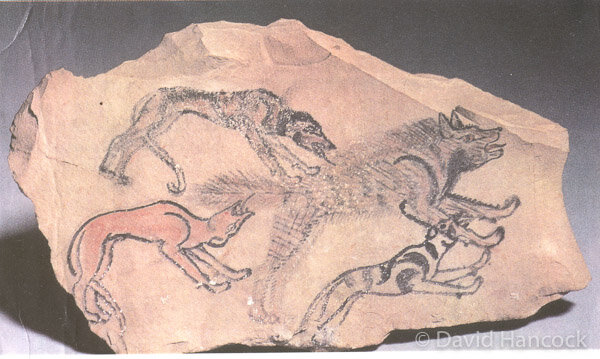This detailed image features a rough-edged rock with a light tan to pinkish-brown hue, suggesting a possible archaeological or ancient origin, potentially from a cave or historical excavation site. Intriguingly, the rock displays a series of intricate etchings or drawings depicting various canines, likely resembling wolves, dogs, hyenas, or coyotes. There are four prominently visible animals on the rock: one with a distinctly furry appearance, another adorned with stripes, a third characterized by a solid brown color, and a fourth marked by gray tones. A unique brush-like pattern gives texture to the drawings. Notably, in the bottom left corner, there is a striking depiction of a red, devilish-looking dog, while the bottom right bears the signature "David Hancock," presumably attributing the artwork or photograph to this individual. The rock's etchings offer a captivating glimpse into artistically represented wildlife, set against a gray background.